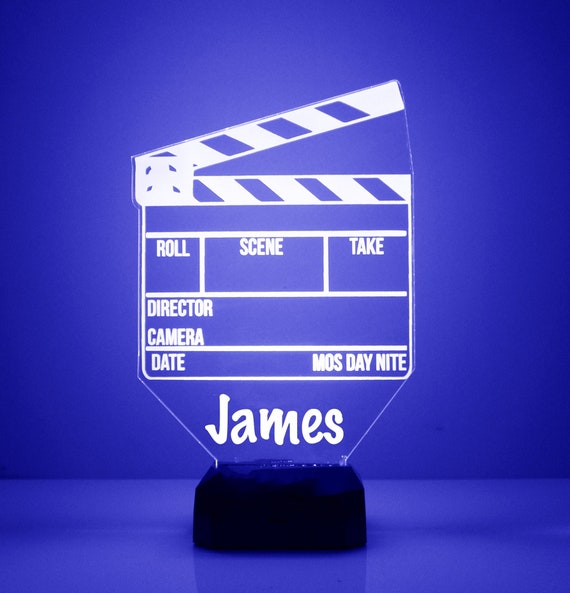The image depicts an award prominently displayed on a blue table with a solid dark blue background, illuminated by a spotlight that casts shadows around it. The award, made of lucite, is crafted into the geometric shape of a movie clapperboard, a tool traditionally used in filmmaking to mark scenes. The top section of the award features a detailed white etching of a clapperboard with labeled boxes for "Role," "Scene," "Take," "Director," "Camera," "Date," "MOS," "Day," and "Night." Below these boxes, in a large, stylized font, the name "James" is inscribed. The award sits on a black base and the overall composition of the image suggests it is a specialized accolade, possibly recognizing James's contributions to the film industry. The color palette of the image is dominated by shades of blue and black, with the bright blue backdrop giving a striking contrast to the clear lucite and dark base of the award.